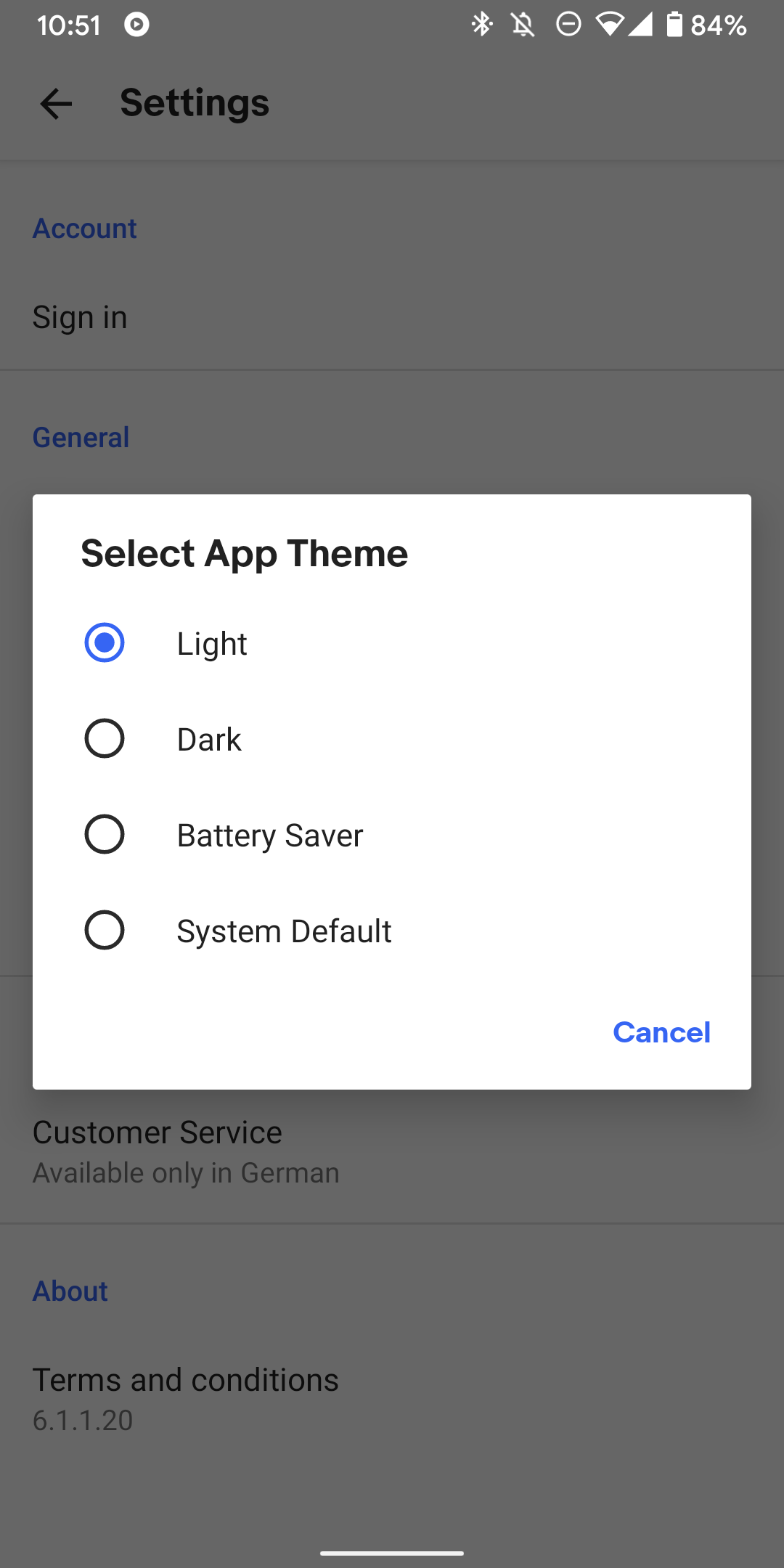Screenshot of a smartphone settings page displaying a selection menu for themes. The screen has a gray, transparent overlay with a white box on top. Inside the box, written in black text, are options related to theme selection. The currently selected theme is "Light," with additional options for "Dark," "Battery saver," and "System default," along with a "Cancel" button. The smartphone status bar shows a timestamp of 10:51, Bluetooth enabled, sound muted, Wi-Fi connected, and a battery level at 84%. Below the white box, the settings menu includes options for "Account," "Sign-in," "General," and a note indicating "Customer service available only in Germany." Additional sections are "About," "Terms and Conditions," and a version number "6.1.1.20." The page also features a back button represented by a left-facing arrow to navigate to the previous screen.